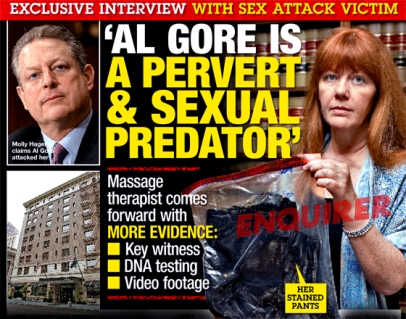This image is designed to resemble the sensationalistic front cover of a tabloid magazine, featuring a bold and striking layout. At the very top, a red bar with white text announces an "Exclusive interview with sex attack victim," followed by yellow text emphasizing the victim's statement. Dominating the center of the cover, larger white and yellow text proclaims, "Al Gore is a pervert and sexual predator," with additional red text likely presenting further lurid details, though it is illegible. There’s a photo of Al Gore in the top left corner, portraying him in a black jacket, white button-up shirt, and tie, with a clean-shaven face and short hair. Below this, an image of a large building in a city is placed.

On the right side of the cover, a woman with red hair, dressed in a blue shirt and wearing a bracelet on her left arm, is prominently displayed. She holds a sealed Ziploc bag, which a yellow speech bubble identifies as containing "her stained pants." Above her, the magazine's title, "Inquirer," is prominently displayed in red lettering. The background behind the woman resembles a library of law books.

Below the main headline, additional white and yellow text informs readers that a "Massage therapist comes forward with more evidence," listing "key witness, DNA testing, video footage" in bullet points. The colors used throughout the cover include a striking combination of red, white, yellow, black, light blue, gray, tan, and orange, contributing to the overall sensationalist and eye-catching design typical of tabloid journalism.